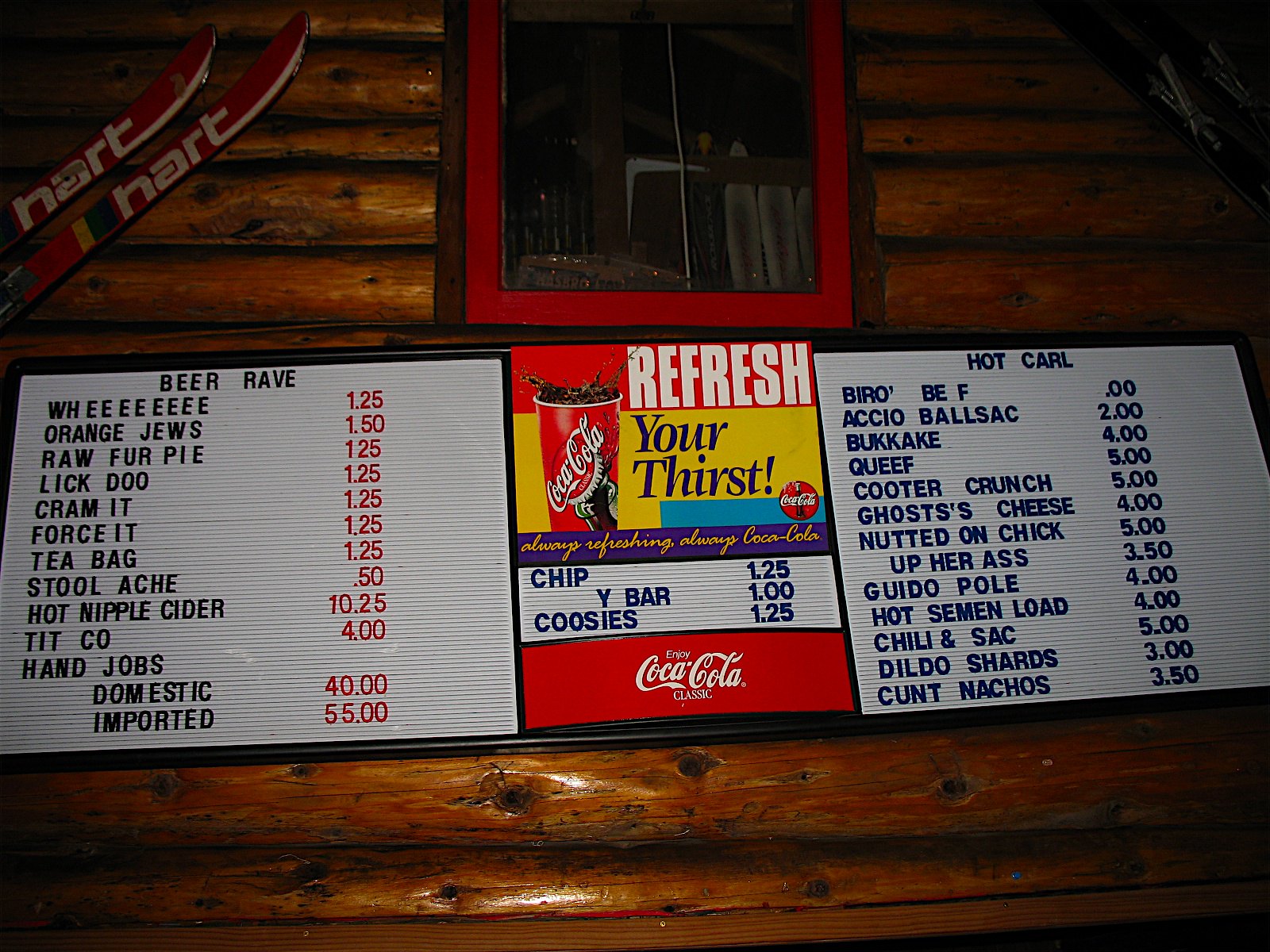In this photograph, we see an interior designed to mimic the rustic charm of a cabin, although it is inside a restaurant. The focal point is a log wall adorned with a framed mirror, reflecting the cabin-like decor. The restaurant has cleverly embraced the theme, giving diners a cozy, woodland experience. Centered on this log backdrop is a prominent Coca-Cola advertisement. The ad features an image of a refreshing Coca-Cola cup with the beverage splashing out, accompanied by the slogan "Refresh Your Thirst." Below this, the ad lists "Chips e Barcooses" with prices of $1.25 each. 

The menu is divided into two sections. The left-hand side is titled "Beer Rave" and lists creatively named drinks, including "Wee," "Orange Juice," "Raw Fur Pie," "Lick Dew," "Cram It," "Force It," "Tea Bag," "Stool Ake," "Hot Nipple Cider," "Titco," "Handjobs," and "Domestic Imported."

On the right-hand side, the menu section titled "Hot Carl" lists food items with equally whimsical and provocative names. These include "Biro Beef," "Asio Ball Sack," "Buckack," "Queef," "Cooter Crunch," "Ghost's Cheese," "Nutted on Chick," "Up Her Ass," "Guido Pull," "Hot Semen Load," "Chili and Sack," "Dildo Shards," and "Cunt Nachos," with prices ranging from $1.25 to $55.

A light emanates from behind, casting a warm glow that reflects off the cabin logs, enhancing the cozy, intimate atmosphere of the restaurant.